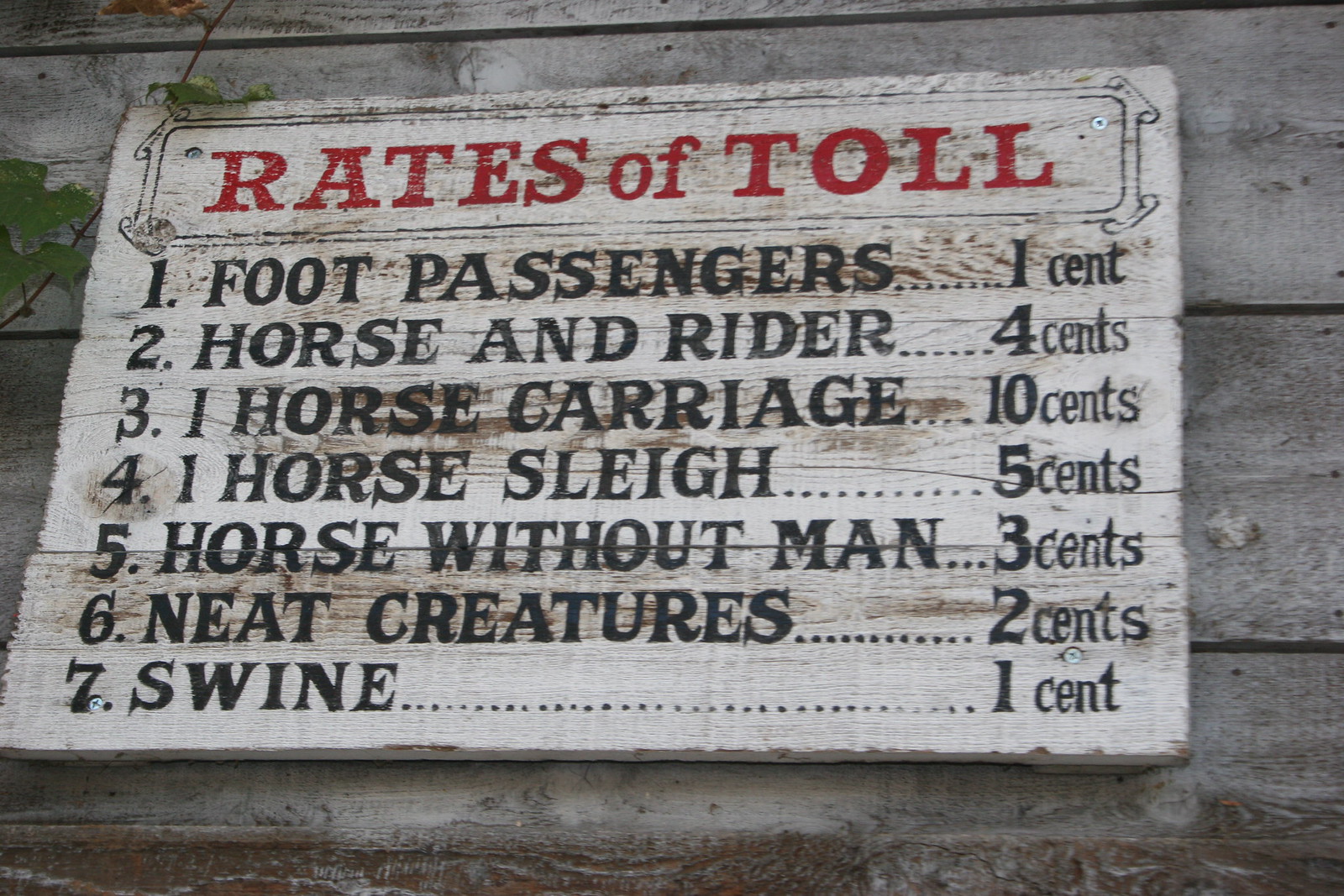This color photograph features a weathered, white-painted wooden sign, screwed into a gray, slatted wooden wall. The sign, bordered in black, prominently displays "RATES OF TOLL" in bold red capital letters at the top. Below the heading, a list enumerates various toll rates in slightly faded black type:

1. Foot passengers: 1 cent.
2. Horse and rider: 4 cents.
3. One horse carriage: 10 cents.
4. One horse sleigh: 5 cents.
5. Horse without man: 3 cents.
6. Neat creatures: 2 cents.
7. Swine: 1 cent.

The sign's appearance suggests it has been exposed to sunlight, giving the wood a lighter, faded brown hue. The detailed and slightly worn text remains clear enough to convey its historical significance.